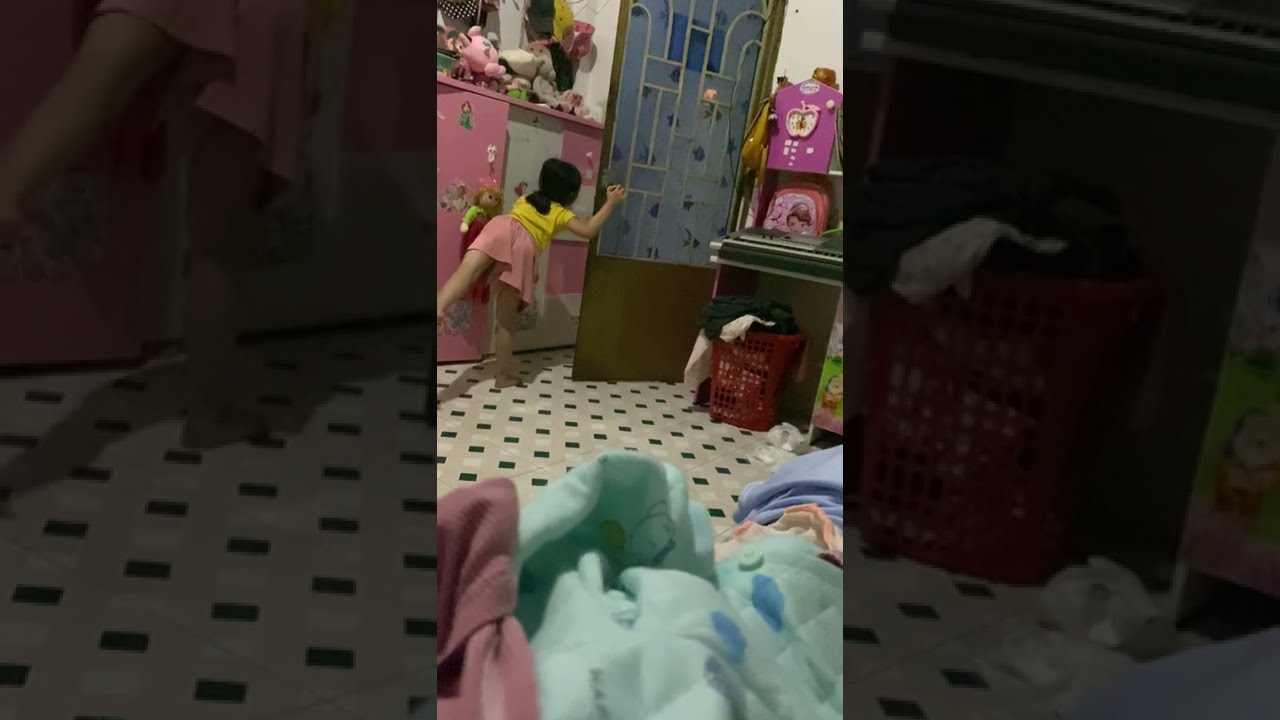This photograph captures the interior of a room, likely a child's room, with a vintage or 60s style ambiance, featuring elements that might suggest it's located in regions like China or the Bay Area. The scene is divided into three vertical sections, with the left and right sections being semi-transparent, magnified versions of the central part. The main focus is a small girl with black hair in a ponytail, wearing a yellow shirt and a pink skirt. She is leaning forward on one leg, her other leg extended behind her, and is holding onto the doorknob of a door adorned with a light blue rectangular design. 

The floor beneath her is a black and white tile floor with a pattern of black diamonds on white tiles. In the background, to the left of the girl, there are pink and white cabinets with household items on top, and a desk with a red laundry basket filled with clothes underneath it. The laundry basket is overflowing with green, white, and possibly other color clothes. In the foreground, piles of pink, light blue, and possibly peach-colored blankets and garments are visible, adding to the lived-in feel of the room.